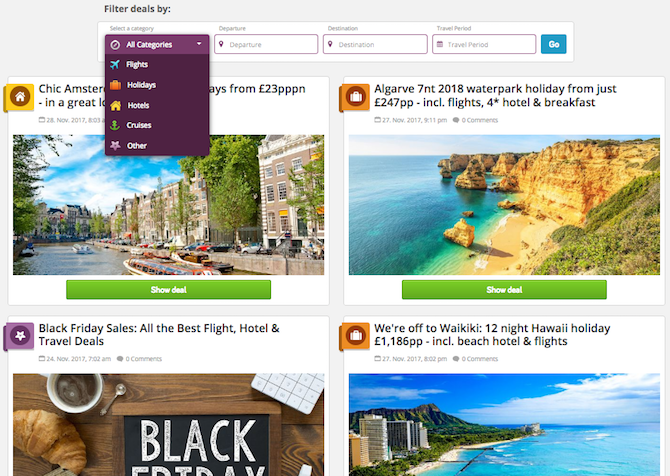The image showcases a travel booking website designed to help users find deals on flights, hotels, holidays, and cruises. At the top of the webpage, there's a filtering option with a drop-down menu labeled "Filter Deals By" where users can select categories such as Flights, Holidays, Hotels, and Cruises. Adjacent to the drop-down menu are input boxes for selecting the departure date, destination, and the duration of travel, followed by a prominent blue "Go" button. 

Below the filters, four travel deal options are displayed. The first option, partially obscured by the drop-down menu, appears to be a deal for Amsterdam, featuring an image of buildings lining a canal with boats and trees. A green horizontal bar with the text "Show Deal" is just beneath the image. 

To the right of this, there is a water park holiday deal, represented by an image of water and cliffs, also accompanied by a "Show Deal" button.

The next two deals are partially cut off but are still visible. The third deal is a Black Friday special, which highlights the best flight, hotel, and travel deals, illustrated by an image of a coffee and croissant on a table. It is marked with another banner stating "Black Friday."

The fourth and final deal promotes a trip to Waikiki, Hawaii, featuring an image of the shoreline, numerous buildings, and the clear blue waters, enticing the viewer with a glimpse of paradise.